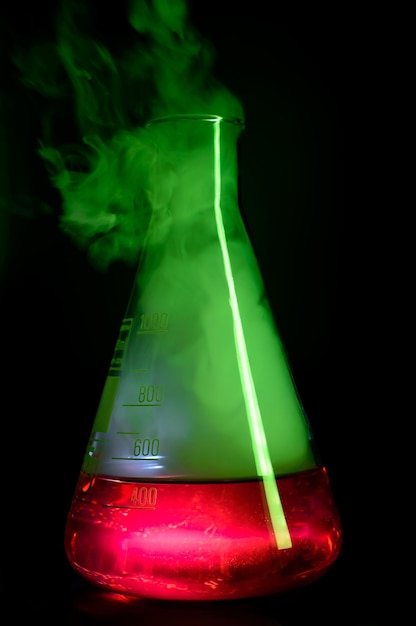This photograph depicts a Halloween-themed chemistry scene, centered on a classical Erlenmeyer flask made of glass. The flask is positioned against a completely black background, accentuating the striking colors within. At the base of the flask, a luminescent scarlet red liquid rests, filling the space between the 400ml and 600ml marks. Above this red liquid, the contents transition into a vibrant emerald green, from which a thick plume of smoke emanates and billows upwards, suggesting an active chemical reaction akin to those found in a mad scientist's lab. The beaker's measurements are clearly visible along its left side, and it appears to be illuminated from behind, giving it a glowing effect that highlights the dramatic contrast between the red liquid and the green smoke. A stripe of light enhances the side of the beaker, contributing to the overall eerie and scientific atmosphere of the scene.